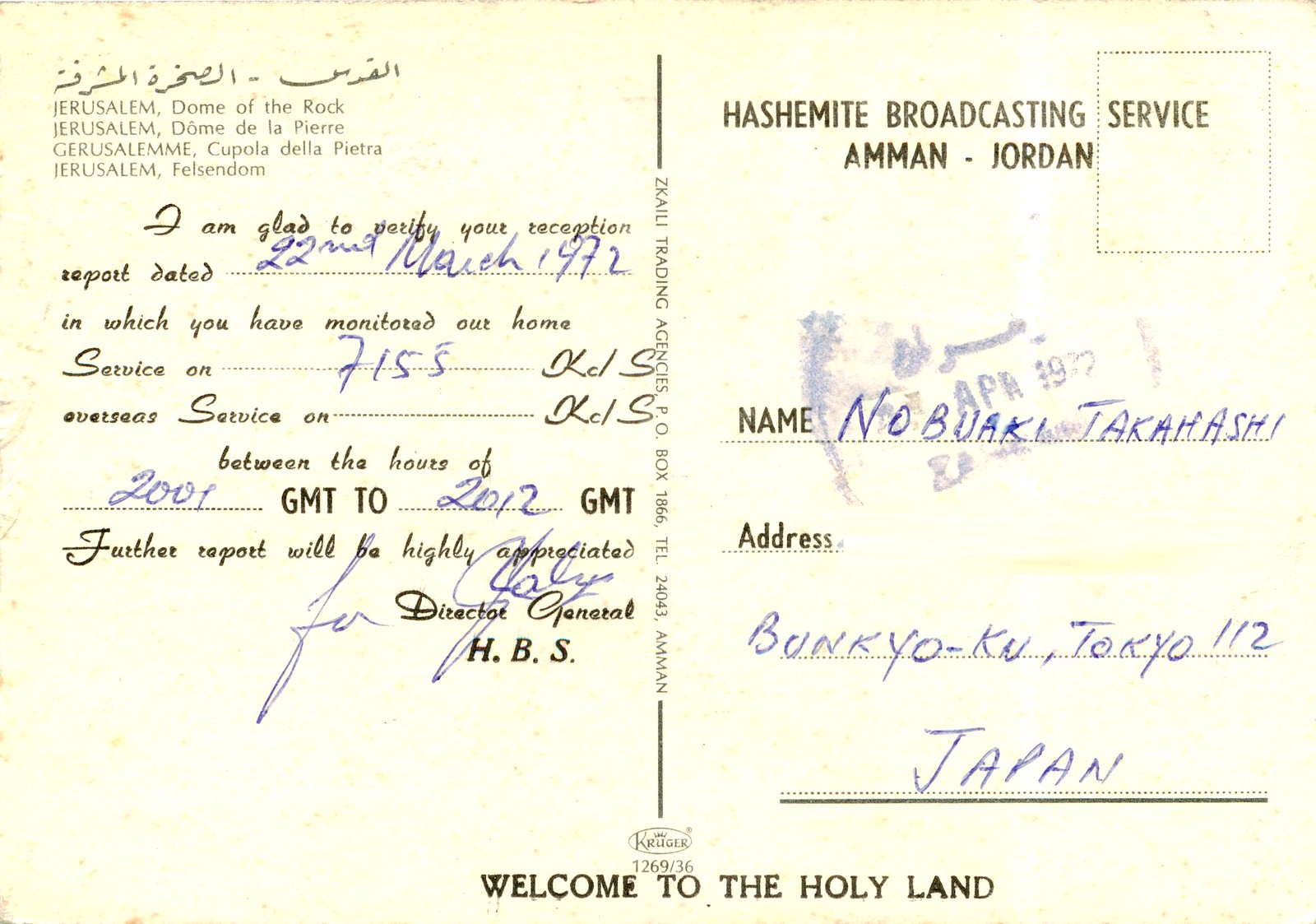This is an image of the back of an old postcard styled as a religious broadcast verification card. The top right corner of the card is printed with "Hashimite Broadcasting Service, AMMAN, Jordan." The vertical line dividing the postcard reads, "Zycali Trading Agencies, PO Box 1866, Telephone 24043, AMMAN." The bottom of the postcard is printed with the words "Welcome to the Holy Land."

To the left of the line, various historical names for the "Jerusalem Dome of the Rock" are printed in multiple languages - "Jerusalem Dome of La Pierre," "Jerusalem Cupola Della Pietra," and "Jerusalem Felsendron." Below this, a handwritten message in blue ink states: "I am glad to notify your reception report dated 22nd March 1972, in which you have monitored our home service on 7155 KCLS between the hours of 2001 and 2012 GMT. Further reports will be highly appreciated." It is signed, "Director General H.B.S."

On the right side of the line, the printed text "Name" and "Address" prompts are filled in with the handwriting "Nobuaki Takahashi, Bonkyo-Ku, Tokyo 112, Japan," respectively. The card confirms the individual's report of monitoring specific broadcast frequencies, likely indicating it's a thank-you note for receiving reception feedback on a shortwave radio broadcast. The printing is in black ink, but there is no stamp affixed to the postcard.